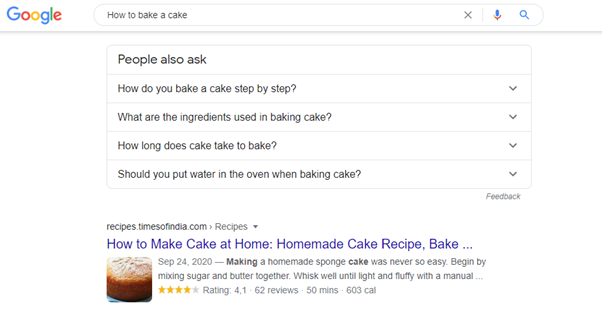A screenshot of a Google search results page is depicted, showcasing information on "how to bake a cake." The layout is centrally justified with a clean, white background adorned with predominantly black text. Color accents stem from the recognizable Google logo positioned at the top left, featuring its signature blue, red, yellow, and green hues. 

At the top center, the user’s query, "how to bake a cake," is visible in the search bar. Adjacent to this, towards the right, are functional icons including an 'X' for clearing the search, a microphone for voice input (speech-to-text), and a magnifying glass for initiating a new search.

Beneath the search bar, a section labeled "People also ask" presents a series of related questions: 
1. "How do you bake a cake step-by-step?"
2. "What are the ingredients used in baking a cake?"
3. "How long does cake take to bake?"
4. "Should you put water in the oven when baking a cake?"

Further down the page, the first search result from timesofindia.com titled "How to bake a cake at home, homemade cake recipes" appears, indicating its relevance to the user's query.